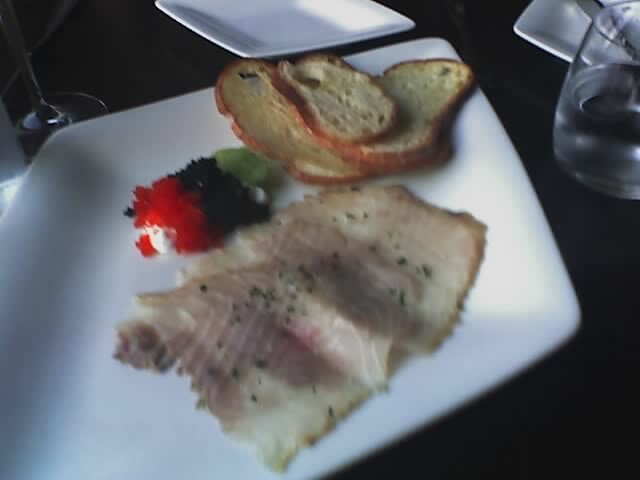The image depicts a somewhat sparse and disorganized arrangement of food on a countertop covered with a black tablecloth. At the center, there is a small, square, white plate featuring a few pieces of thinly sliced, toasted bread with darker brown edges. Beside the bread is a thinly sliced, pale-colored piece of meat, potentially deli-style or fish; its pinkish center and slightly fatty texture suggest it could be fish with visible lines in the meat. Accompanying these items is a small trio of colorful spreads or toppings, likely caviar or similar delicacies, in red, black, and green hues. To the left of the main plate, there appears to be a jar of water, and another clean white plate is present on the table. The lighting within the image is quite dim, casting a dark ambiance around the countertop, making it difficult to discern additional details or items beyond the main plate setup. The overall impression is that the meal is a small, possibly gourmet dish, perhaps intended for a special event or tasting.